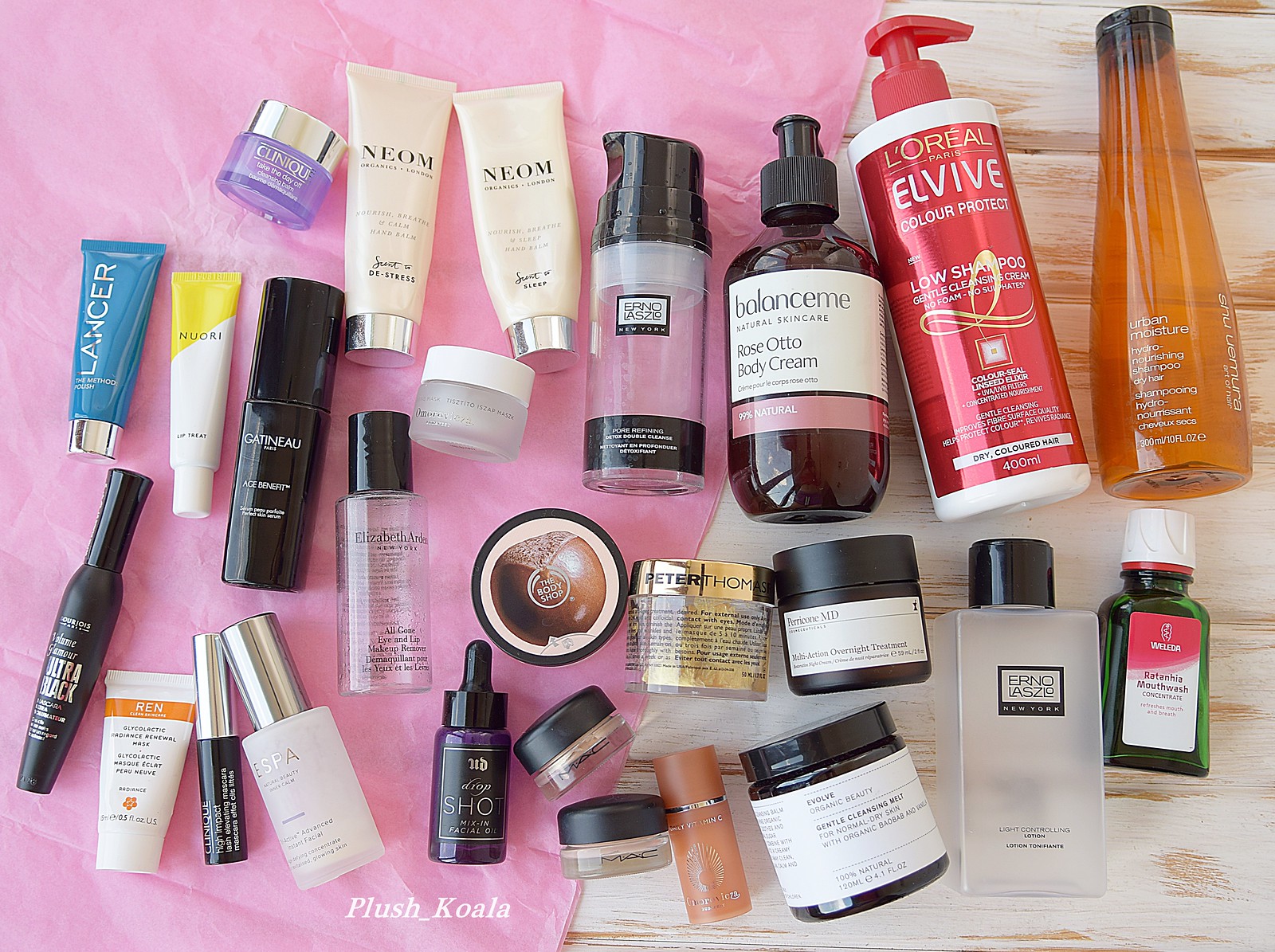The image showcases an extensive variety of women's beauty and cosmetic products meticulously arranged on what appears to be a white wooden table, possibly made of pine or beech. Over half the table is adorned with a pink piece of tissue paper, providing a delicate backdrop for the collection. An image credit in white lettering at the bottom reads "plush_koala."

There are approximately 20 beauty products of different sizes and types, organized in rows that form gentle waves across the table. Here's a detailed breakdown of the items:

1. **Top Left**: A small container with a silver lid and purple translucent base labeled "Clinique Take the Day Off Cleansing Balm."
   
2. **To the Right**:
    - Two nearly identical lotion bottles in pale cream color with silver bases, labeled "Neom Organics London." One is "Secret Destress," and the other is "Secret Sleep," likely both hand creams.

3. **Next**: 
    - A serum bottle with a black pump and a black label named "Erno Laszlo New York Pore Refining Double Cleanser."

4. **To the Right**: 
    - A clear bottle with a black pump and brown contents, labeled "Balance Me Natural Skincare Rose Otto Body Cream." Contains text in French and claims to be 99% natural.

5. **Further Right**: 
    - A white bottle with a red pump and a prominent red label, part of the L'Oreal Paris Elvive line. It reads "Color Protect Low Shampoo, Gentle Cleansing Cream, No Foam, No Sulfates, Color Seal, Linseed Elixir," for dry colored hair, 400 ml.

6. **Directly Right**: 
    - An orange bottle resembling a melted vase and wine bottle with the label "Urban Moisture Hydro-Nourishing Shampoo for Dry Hair," seemingly from a brand called "Bunwin Nus."

**Second Row**:
1. **Left**: 
    - A blue bottle labeled "Lancer The Method Polish."

2. **Adjacent**: 
    - A small tube resembling chapstick, marked "Nuori." It is primarily cream-colored with a yellow diagonal slant on the top half.

3. **Next**: 
    - A long black bottle labeled "Gatineau Paris Age Benefit."

4. **Further Right**: 
    - A black bottle reminiscent of a hand sanitizer, labeled "Elizabeth Arden New York All Gone Eye and Lip Makeup Remover," with the same text in French.

5. **Adjacent**: 
    - A smaller frosted glass bottle with a white lid, difficult to read the label but smaller than the Clinique container.

6. **To the Right**: 
    - A bottle featuring a coconut image with "The Body Shop;" the product type is indiscernible.

7. **Next**: 
    - A jar labeled "Peter Thomas Roth," featuring pale gold flakes, though the rest of the text is hard to read.

8. **In Sequence**: 
    - A smaller black canister labeled "Perricone MD Multi-Action Overnight Treatment."

9. **Far Right**: 
    - A frosted glass bottle with a black lid labeled "Erno Laszlo New York Light Controlling Lotion."

10. **Furthest Right in Row**: 
    - A green bottle labeled "Weleda Ratanhia Mouthwash Concentrate."

**Bottom Row**:
1. **First Left**: 
    - A black mascara marked "Ultra Black."

2. **Next Right**: 
    - A white bottle resembling lotion labeled "Ren Clean Skincare," some sort of renewal mask.

3. **Subsequent**: 
    - Another mascara from Clinique.

4. **Further Right**: 
    - A frosted white bottle with a silver lid labeled "Espa," the size of a nail polish bottle.

5. **In Sequence**: 
    - A small dropper bottle labeled "Drop Shot Mix-In Facial Oil."

6. **Next**: 
    - Two clear bottles, presumably containing MAC makeup.

7. **Toward the End**: 
    - An orange bottle, squash-like in design, related to Vitamin C.

8. **Last Item**: 
    - A product labeled "Evolve Organic Beauty Gentle Cleansing Melt."

The collection indicates a keen interest in skincare, housing both high-end luxury items and more affordable products.